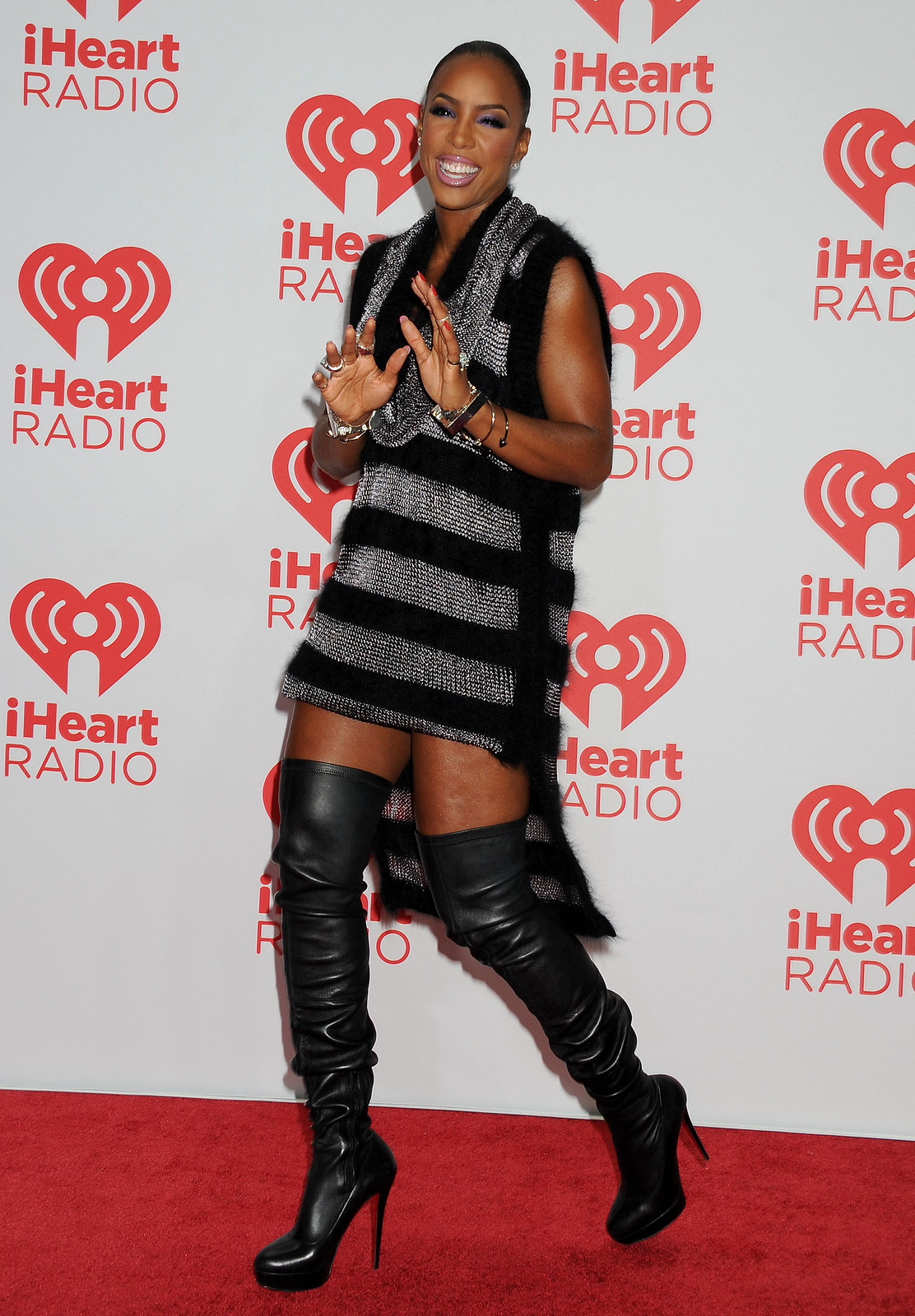Kelly Rowland, a member of Destiny's Child, is captured in this vibrant photograph standing on the red carpet in front of an iHeartRadio backdrop featuring repeated brown logos with a distinctive red heart. She beams with a big, vibrant smile, showcasing her full professional makeup. Kelly is dressed in a sleeveless shift dress adorned with alternating mesh silver and cashmere-like black stripes, along with a slouchy scarf or loose collar line. On her wrists, she displays several silver bracelets, complemented by multiple diamond rings on her fingers and small stud earrings. Adding height to her look, she wears thigh-high black leather stiletto boots. The image prominently captures her joyful and dynamic presence in an 8-inch tall by 5-inch wide frame.